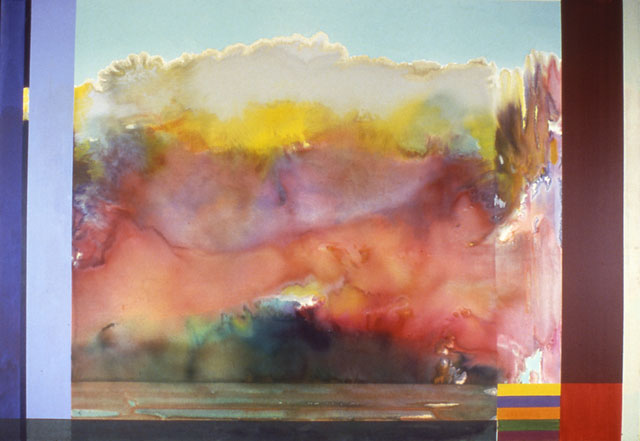The image captures a watercolor painting with an abstract composition of layered colors resembling clouds and terrain, showcased against a blue sky. The various hues blend seamlessly, creating a fantastical landscape.

Starting from the bottom, the painting features a tan and dark brown layer that could suggest a distant terrain with indistinct, small figures. This layer extends horizontally towards the left and right. Above this, there's a blend of teal and dark blue, giving way to a large mass of orange and red. Central to the composition, the blue and green sections merge, bordered by a prominent expanse of light red that rises to the midway point.

Further up, a pinkish-purple section interspersed with patches of blue merges gradually into yellow. Toward the upper layers, greenish-black hues interlace with the yellow. The painting culminates in a topmost layer of creamy vanilla white against a backdrop of a blue sky.

On the right side of the painting, the frame shows a gradient of dark red to bright red, while the left side features light and dark blue. The overall impression is a grainy, splotchy texture typical of watercolor, evoking an abstract field of colors that may represent an ethereal sky filled with dynamic, shifting clouds.